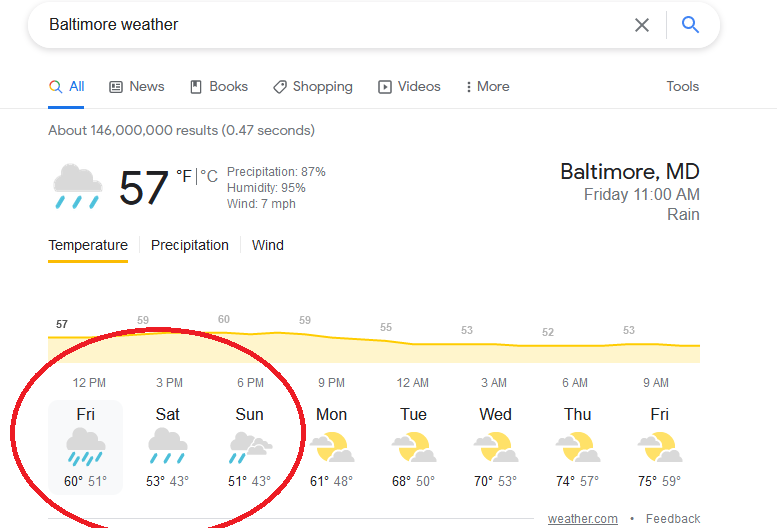This image is a detailed screenshot of a Google search results page for "Baltimore weather." The background is white, and across the top, the search bar displays the query "Baltimore weather" in black text. Below this, tabs labeled "All," "News," "Books," "Shopping," "Videos," "More," and "Tools" are visible, with the "All" tab currently selected. Directly beneath these tabs, it states "About 146,000,000 results (0.47 seconds)" in black text.

On the left side, there is an image of a gray cloud with three raindrops, indicating the current weather. Next to this, it shows the temperature as 57°F, with additional details such as 87% precipitation, 95% humidity, and wind at 7 mph. Below this information, the weekly weather forecast is displayed.

The forecast starts with Friday, showing the weather for each day of the week. Friday, Saturday, and Sunday are highlighted with red circles, indicating rainy conditions with temperatures of 60°F, 53°F, and 51°F respectively. The remaining days of the week—Monday, Tuesday, Wednesday, Thursday, and the following Friday—are depicted as sunny with partial clouds, with temperatures ranging from 75°F to 61°F.